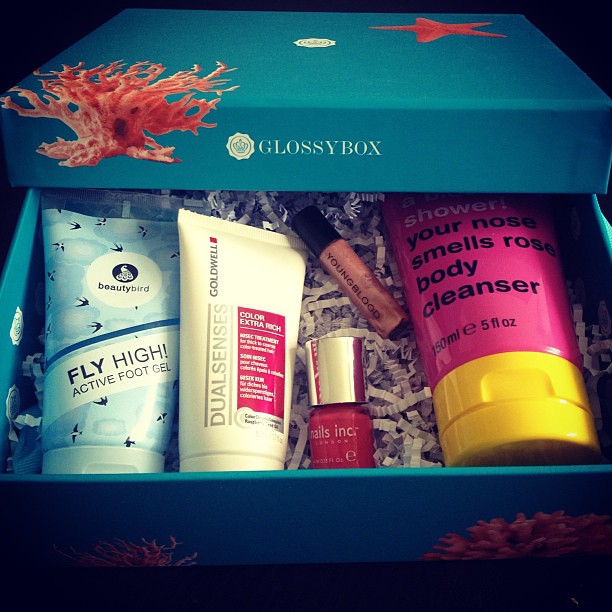The photograph features a partially opened, blue rectangular gift box with a lid that reads "Glossy Box." The box sits against a black background and is adorned with decorative elements such as a pink starfish and some pinkish algae or sponge in the corners, adding a maritime theme. Inside, the box contains crinkly white shredded paper and five cosmetic products arranged neatly. On the left, there is a light blue tube labeled "Beauty Bird Fly High Active Foot Gel." Next to it is a smaller beige tube branded as "Dual Senses Color Extra Rich." A hot pink nail polish bottle with a gold lid and a lip gloss in a light brown shade, marked "Young Blood," are also visible. On the far right, there's a larger pink cylindrical container with black text and a bright yellow lid, partially readable as "Shower Your Nose Smells Roses Body Cleanser." The packaging and layout create a luxurious and aesthetically pleasing presentation of the beauty items.